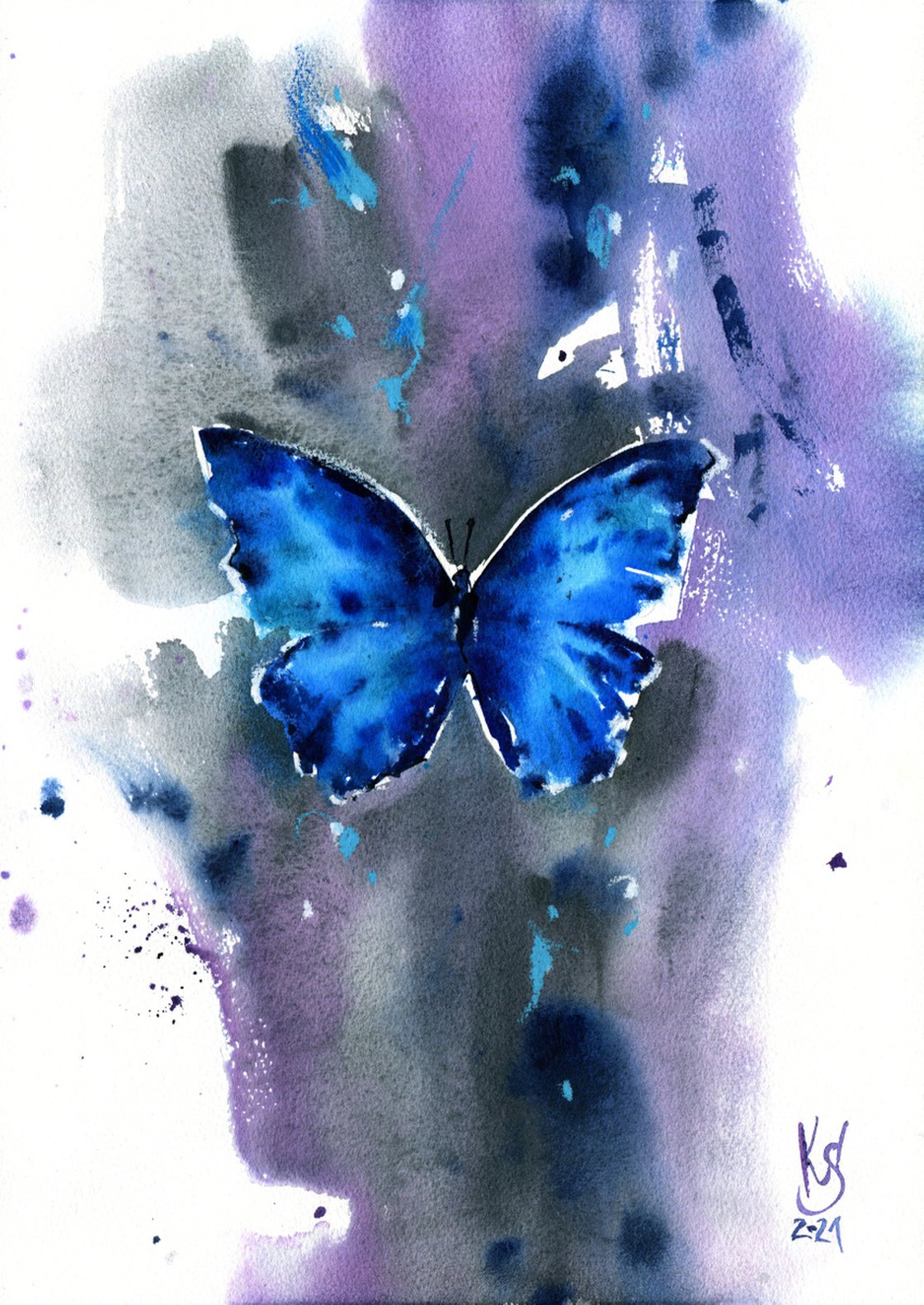This image features an original watercolor painting titled *"Blue Morpho Butterfly"* by the artist Ksenia Selyanko. The painting prominently displays a blue butterfly floating centrally against an abstract background. The butterfly, with its bright blue wings featuring various shades such as royal blue and sky blue, has a dark body and black antennas. The background is a mix of light purple, darker purple, blue, and gray blotches, creating a dynamic and somewhat washed-out effect. The painting lacks a border, blending into the white background of the image, which at times makes it difficult to discern where the painting ends and the background begins. Notably, the lower right-hand corner of the painting is signed "KS" in purple, with the date or edition number "2-29" below it. This signature suggests the work may be an original or part of a limited print series. The overall dimensions of the original artwork measure approximately 11 1/2 inches by 16 1/2 inches.